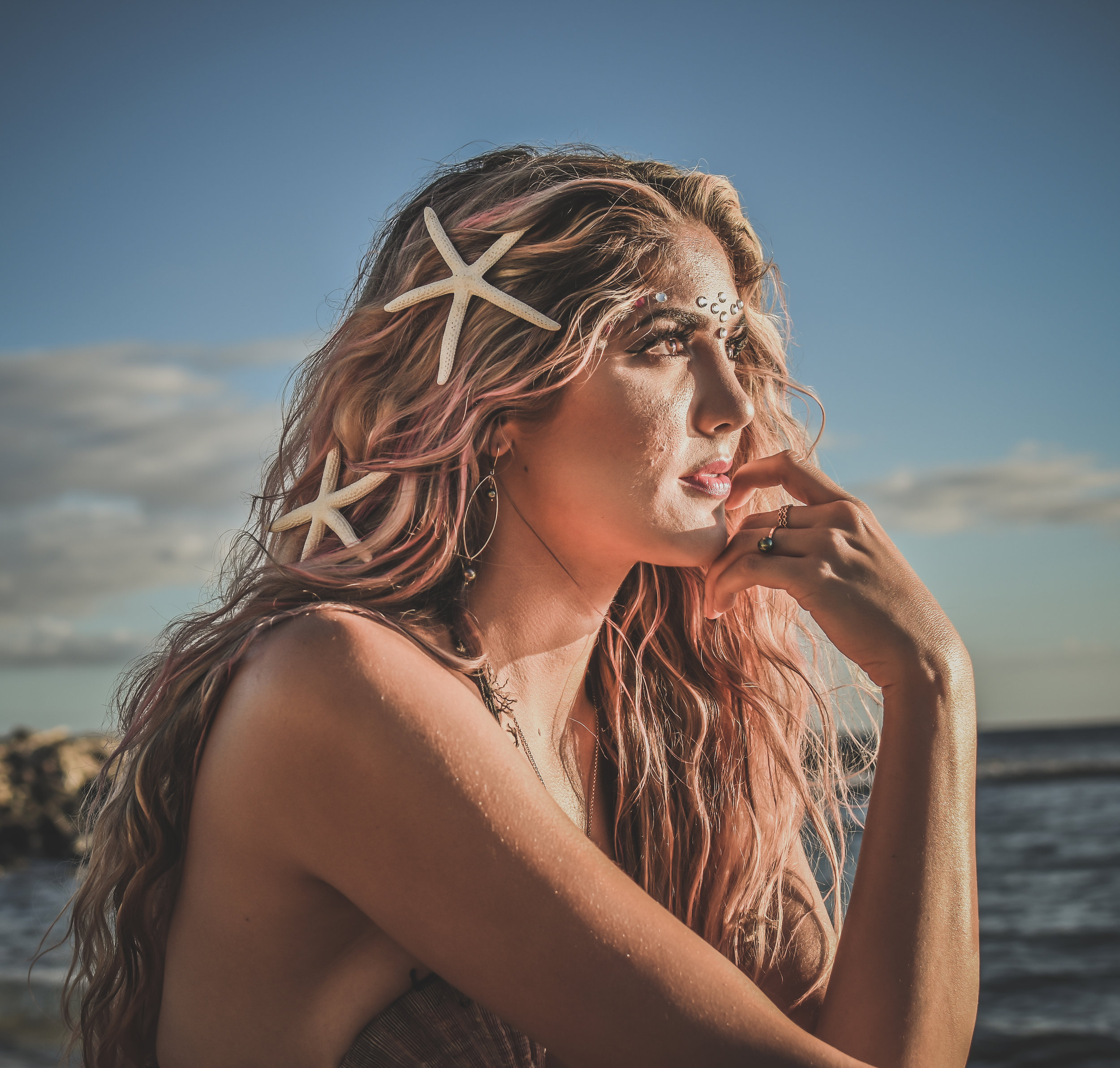The image is a high-quality, square colour photograph of a young woman who appears to be styled as a mermaid. She is seated in the foreground, with her right side closest to the viewer. The image is cropped just below her armpit, showing her torso and part of her right arm angled downwards and off-screen. Her left arm is bent at a 90-degree angle, with her pointer finger touching her lips and her chin.

Her long, wet-appearing hair is predominantly brown with blonde and pinkish highlights. It is draped over her back and front on her left side. Adorning her hair are two large, thin-armed white starfish, placed on the side of her head facing the viewer. She also wears oval hoop earrings with a small bead hanging from each hoop in her right ear.

The woman has a tan complexion and is possibly wearing a bra made of seashells. On her left hand, which is touching her face, she wears rings on two fingers. Across her forehead, above her eyebrows, she has small rhinestones, adding to her mermaid-like appearance. 

She gazes off into the distance with her eyes open, her lips adorned with red lipstick. Behind her, the background features deep blue water on both the left and right sides, with a large beige boulder visible on the left. The sky transitions from darker blue at the top to lighter blue at the bottom, dotted with white and grey clouds primarily on the left side. The sunlight, suggestive of a setting sun, illuminates her face and neck from the side.